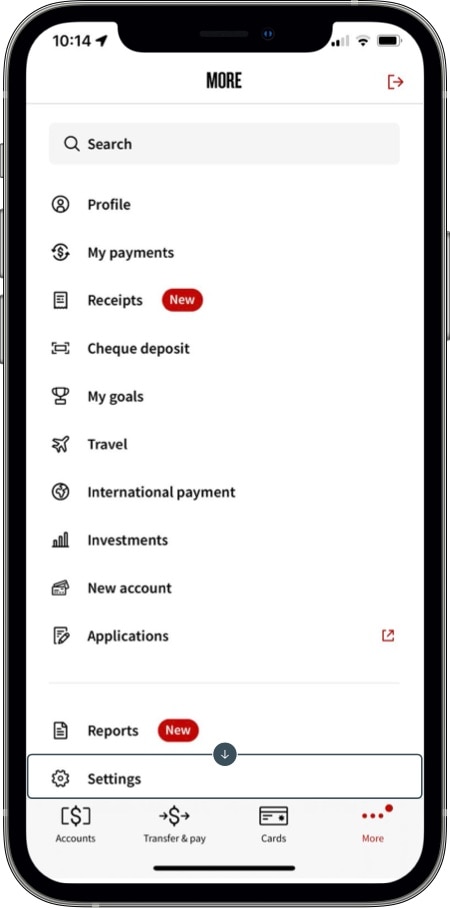This image captures the screen of what seems to be a mobile banking application, likely on an iPhone. At the top left corner, the status bar displays a small black text reading "10:14" accompanied by a location icon. On the right side of the status bar, the battery percentage is visible.

In the center of the screen, an uppercase black text reads "MORE." Directly below it is a search box labeled with the word "Search" in black text and an adjacent search icon.

Beneath the search box is a vertical list of various options, each accompanied by small icons to their left. The options in order are:

1. **Profile**
2. **My Payments**
3. **Receipts** (highlighted with a red oval icon containing the white text "NEW")
4. **Check Deposit**
5. **My Goals**
6. **Travel**
7. **International Payment**
8. **Investments**
9. **New Account**
10. **Applications** (featuring a small arrow icon to the right)

Following this list, another section features an option labeled "Reports," next to which is another red oval icon with white "NEW" text. Below this, "Settings" is listed.

At the bottom of the screen, a navigation bar provides four options: "Accounts," "Transfer and Pay," "Cards," and "More." The first three options are in black text, while "More" is highlighted in red.

Overall, this detailed description ensures that every element on the screen is thoroughly captured and conveyed.